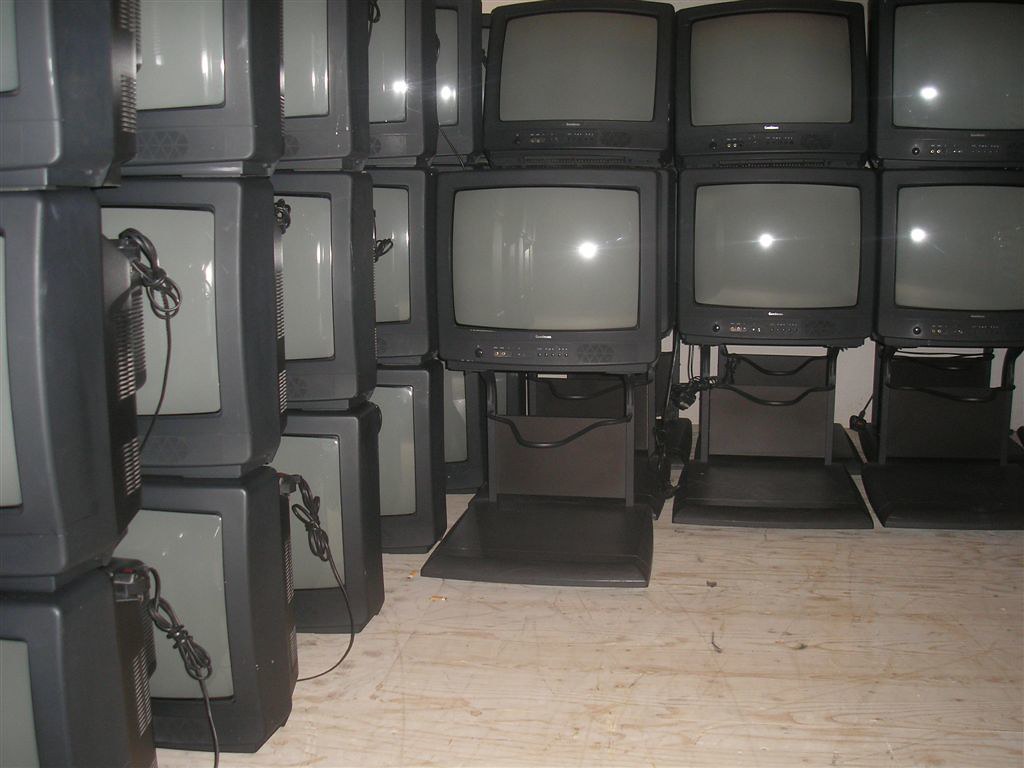This photograph captures a cluttered storage room filled with numerous old CRT TVs, reminiscent of 90s-era bulky box sets with dark gray screens. On the left-hand side of the image, three rows of televisions are stacked three high, extending about five sets deep, with the TVs sitting directly on an unfinished wooden subfloor. The back wall features another set of televisions arranged three across and two high, some perched on black stands. Scattered power cords dangle and are neatly looped for storage. You can see the camera flash reflecting off the TV screens, highlighting the buttons and auxiliary inputs beneath the screens. Although the silver brand names are visible at the center below the screens, the specific names are indistinguishable. The overall scene is a chaotic but organized repository for these nostalgic electronics.